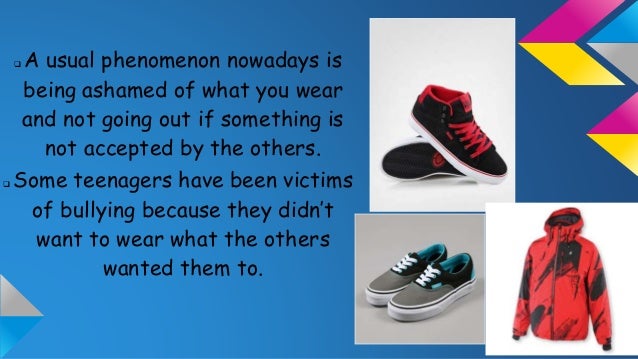The image appears to be part of an advertisement or presentation on the subject of clothing and social pressures among teenagers. The background is a gradient blue, slightly lighter in the center and darker towards the right edge. In the top right corner, there are pink, yellow, blue, and gray arrows. Below the arrows, there are three individual squares each containing an item of apparel.

The first item, in the top right square, is a pair of red and black sneakers with red laces and a red interior. Directly underneath, in the bottom right square, there's another pair of sneakers that are predominantly gray with teal accents on the inside, toe, and heel, with white laces. Adjacent to these, there's an image of a red and black jacket.

On the left side of the image, there is a block of text in a black Comic Sans font that reads: "A usual phenomenon nowadays is being ashamed of what you wear and not going out if something is not accepted by the others. Some teenagers have been victims of bullying because they didn't want to wear what the others wanted them to." This text emphasizes the social issue of clothing-based bullying and societal pressure on teenagers regarding their attire.